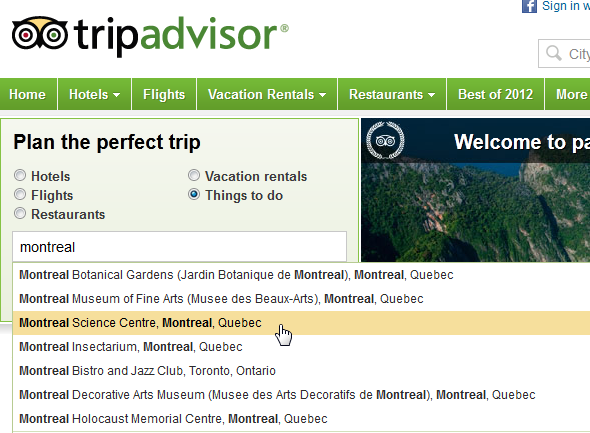This screenshot captures a cropped section from an early 2010s-era website, specifically the top left-hand corner of TripAdvisor. The TripAdvisor logo, featuring the top of an owl's head with large eyes, is prominently displayed at the top left, alongside the site’s name in black and green text. The header is green with white text, offering various drop-down menu options such as Hotels, Flights, Vacation Rentals, Restaurants, and Best of 2012. On the top right, part of a search bar and a Facebook notification button are barely visible. The user is currently on the home page, searching for a trip in Montreal, which has generated a drop-down list of places in Montreal. Highlighted in yellow from this list is the "Montreal Science Centre, Montreal, Quebec," indicating the user's selection.